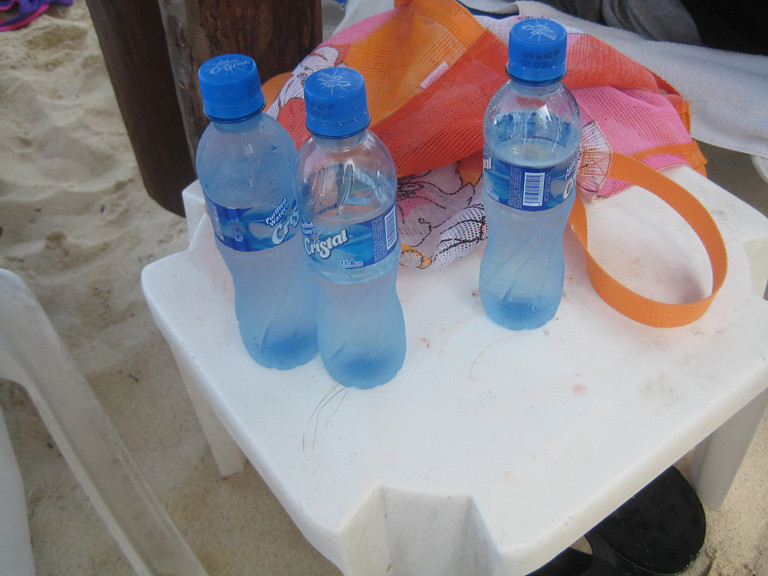In the foreground of the photograph, three small water bottles labeled "Purified Water Cristal" with blue caps are prominently displayed on a white plastic table, situated at a beach. The bottles, appearing cold as if just taken from a cooler, reveal varying levels of water: the left bottle is three-quarters full, the middle one is half full, and the right bottle remains unopened. Surrounding the table, the setup includes details that reinforce the beachside setting: sand is visible below the table, and to the bottom right, a white beach chair's leg can be seen. To the left side of the table sits an orange and pink perforated beach bag adorned with white flowers, collapsed as if empty. In the background, two wooden posts are faintly noticeable, further hinting at the outdoor beach environment.